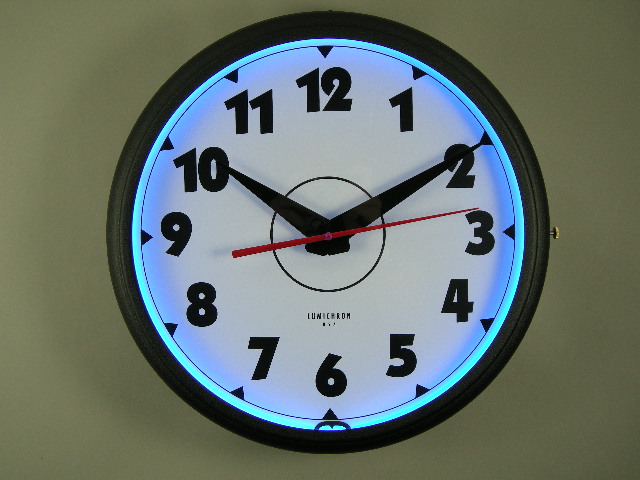This photograph features a round, analog Lumicron clock hanging on a wall, which appears to be painted white. The clock has a striking blue LED illumination around its black rim. The hour, minute, and red second hands indicate the time as 10:10. The clock face displays all numerals from 1 to 12, with black hour markers and hands, contrasted against a light background. A noticeable feature is the LED light providing a blue hue inside the rim. The brand name "Lumicron" is presumed to be printed above the 6 on the clock face. There's a shadow cast by the person taking the picture, which adds depth to the image. Additionally, there's a small knob near the 3, likely used for adjusting the time.